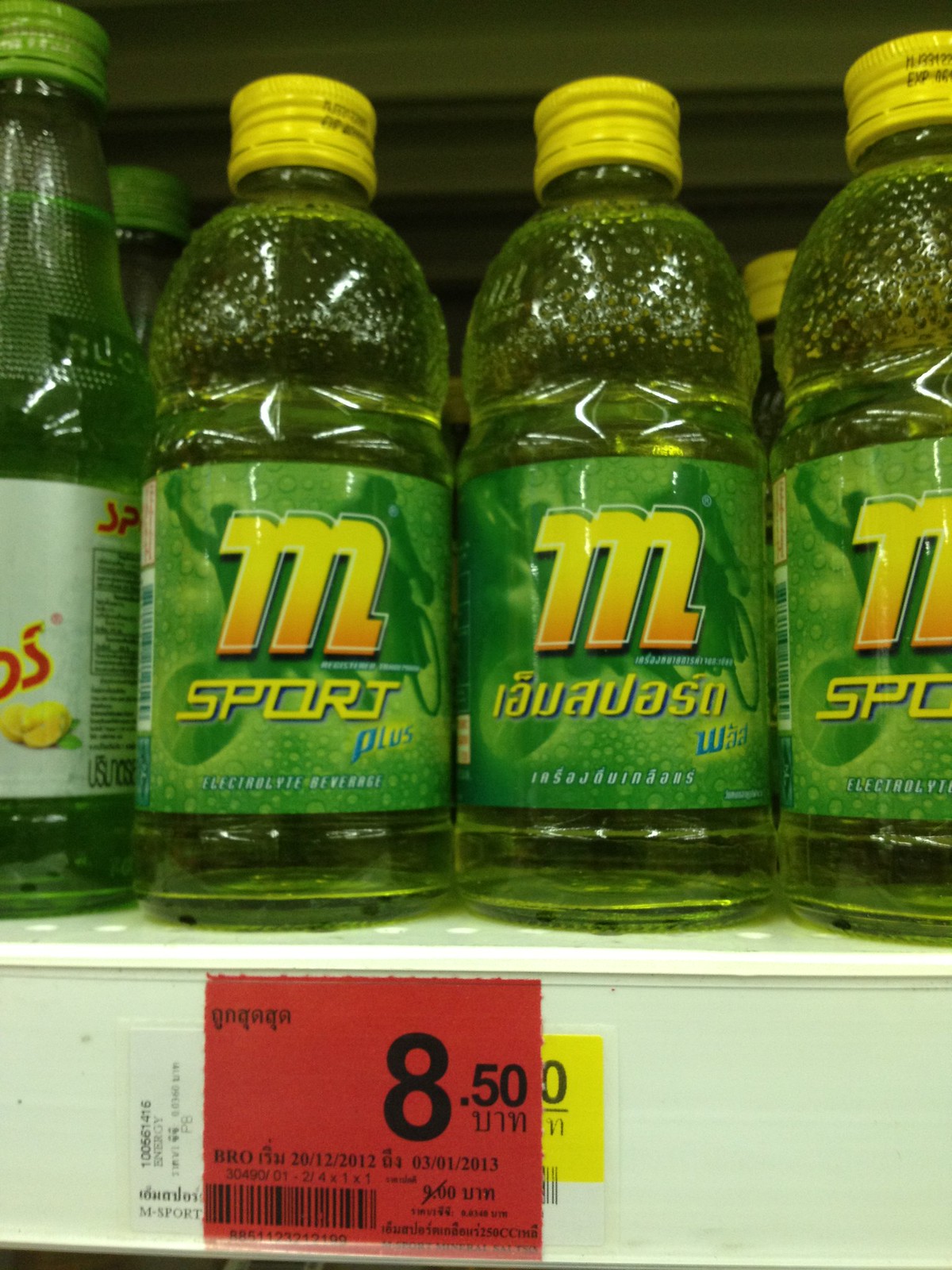This indoor color photograph showcases a shelf in what appears to be a grocery store, prominently displaying bottles of a sports drink. The primary focus is on three green, clear plastic bottles of a beverage labeled "M Sport Plus" with distinctive yellow screw-on caps. The bottles feature a green label with yellow writing, prominently displaying "M" and "Sport Plus," along with additional text in a foreign language. The middle bottle's label is turned, highlighting more of the foreign script. Beneath the bottles on the white shelf is a red and yellow price tag indicating a price of $8.50, suggesting it may be priced in a foreign currency.